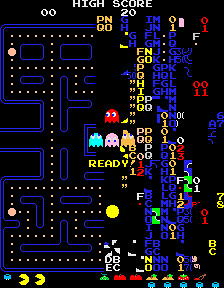The image depicts the screen of the classic video game Pac-Man in vivid detail. The maze is composed of blue LED lines forming various pathways and rectangles. Four colorful ghost characters are visible: a red one, a teal one, a pink one, and an orange one, identifiable as Blinky, Inky, Pinky, and Clyde, respectively. At the top of the screen, the words "High Score" are prominently displayed in white letters, alongside a score of 20. Vertically running letters appear on the screen but do not form recognizable words. At the bottom left, there are two small Pac-Man icons indicating two remaining lives. The screen shows the message "Ready," signaling the imminent start of a new round.